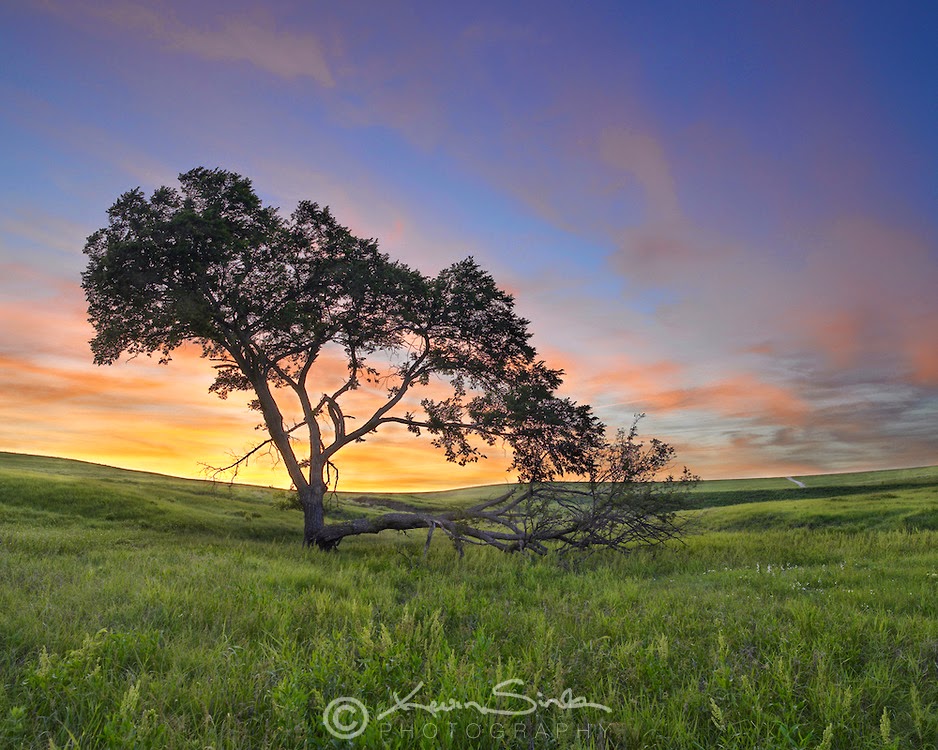The photograph captures a tranquil landscape at dusk, with a vibrant sky dominating the top half of the image. The sky transitions from a deep blue at the very top to a gradient of lighter blues, whites, and finally, rich oranges and dark yellows toward the horizon where the sun is setting. This colorful sky beautifully contrasts the rolling, hilly green field below, which is mostly empty except for a singular tree standing prominently in the center. The tree features two main branches extending upwards and another growing to the right, all covered in dark-colored leaves. A semi-transparent white watermark at the bottom of the image reads "© Kevin Sen Photography," marking the artist's work. This serene and picturesque scene highlights the tree silhouetted against the glowing sky, creating a stunning visual display.